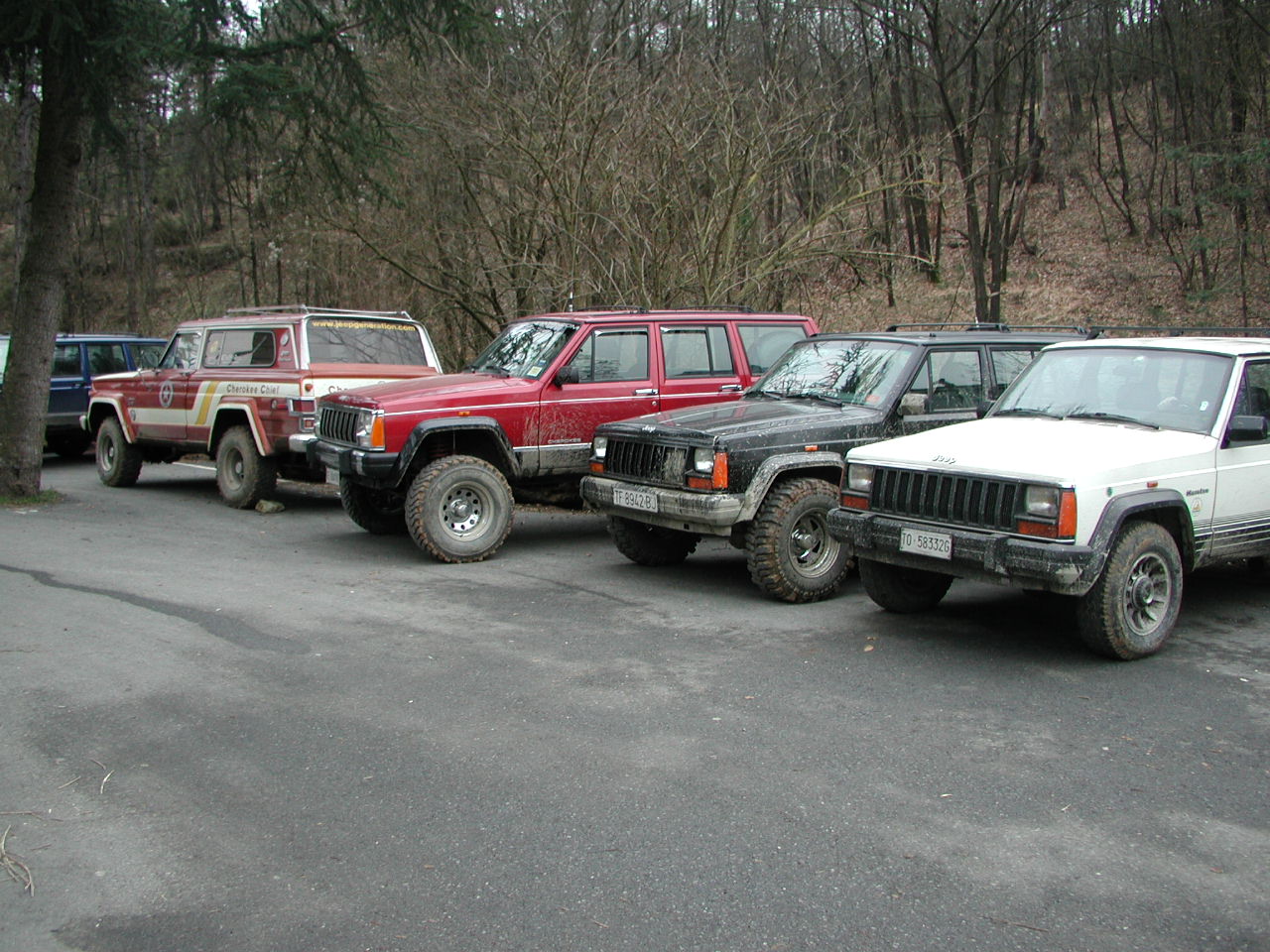This photograph captures a line of five older SUV-style vehicles, reminiscent of Bronco-type trucks or Jeep Cherokees, parked in a parking lot with an asphalt surface that appears wet due to the darker markings. Positioned diagonally, the SUVs significantly stand out against the backdrop of a hilly, wooded area filled with bare, dark trees, characteristic of fall or winter. Starting from the left, the first SUV is a whitish-yellow color, followed by a dark black one with some visible dirt on the hood and tire. The middle vehicle is red, standing slightly taller due to larger tires, and next to it is another red SUV, distinguished by white and yellow diagonal stripes and marked "Cherokee Chief." The last vehicle, only partially visible, seems to be a dark blue color. A notable feature in the left-hand corner is a growing pine tree, adding a touch of green to the otherwise wintry scene.